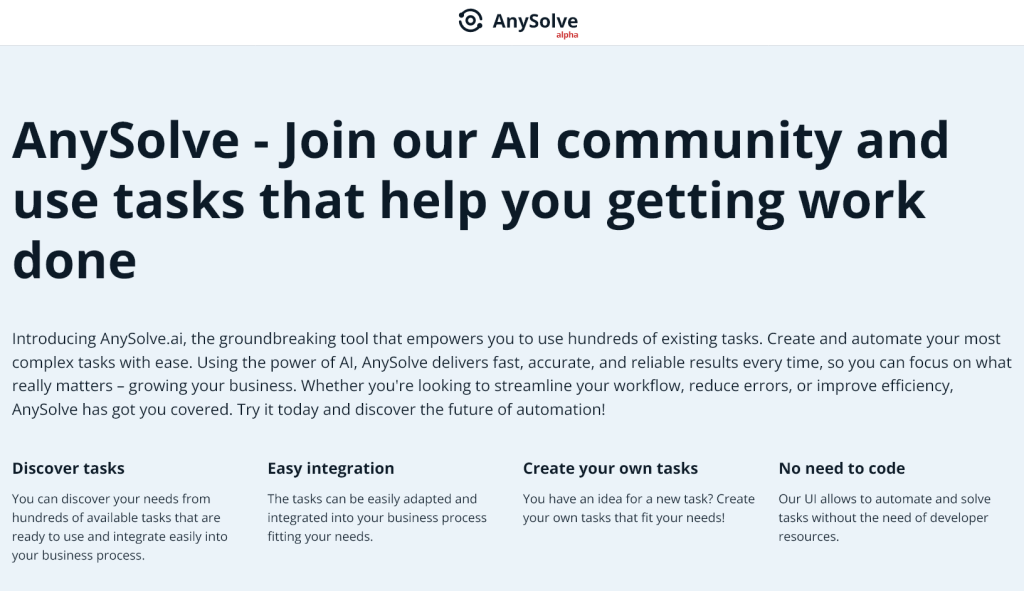The image, sourced from the website AnySolve, prominently features the AnySolve logo at the upper center, with the word "alpha" in red font situated underneath the logo. A tiny alpha symbol is positioned directly below the 'V' and 'E' of AnySolve. Below this, there is a blue square, serving as the background for the main content of the page. 

The title, "Enlarge," is displayed in black font. Beneath the title, the text reads: "AnySolve: Join our AI community and use tasks that help you get work done."

Further down, in smaller font, there is a detailed introduction: "Introducing AnySolve.ai, the groundbreaking tool that empowers you to use hundreds of existing tasks, create and automate your most complex tasks with ease. Using the power of AI, AnySolve delivers fast, accurate, and reliable results every time."

At the bottom of this section, there are four small blurbs, each summarizing different aspects or features of the AnySolve tool.